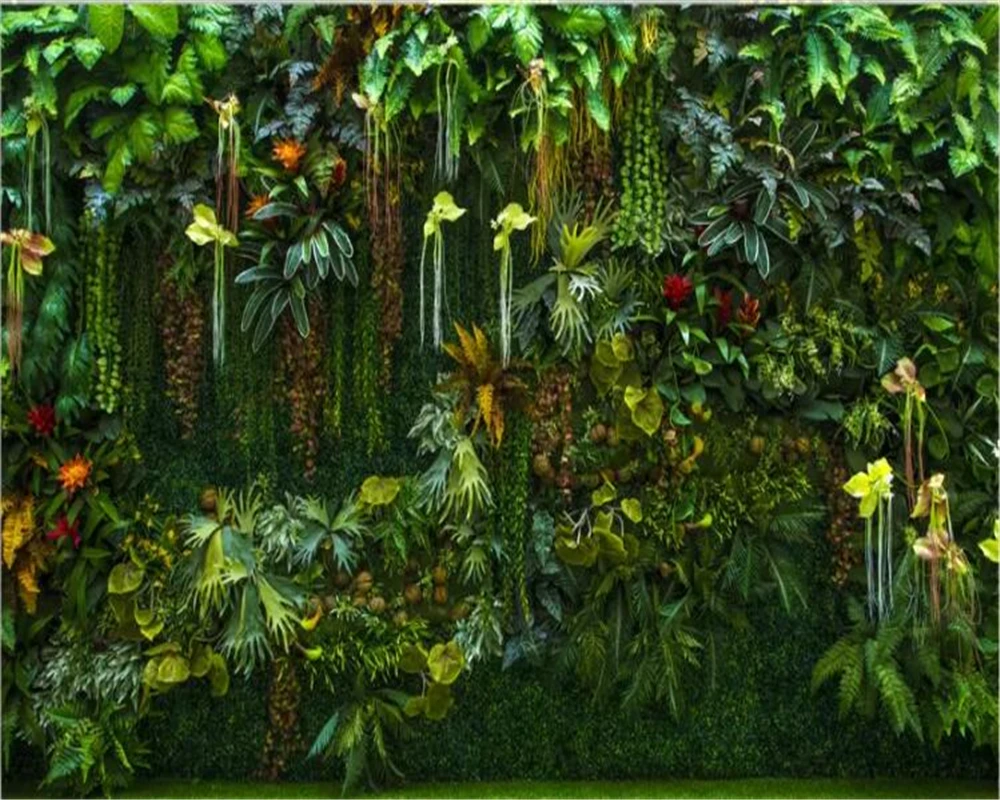This vibrant image showcases a lush, green wall adorned with a diverse array of plants and flowers, potentially evoking the dense atmosphere of a jungle or an artistic green installation. The scene is dominated by various shades of green, ranging from bright to dark hues, interspersed with splashes of red and orange flowers. At the top, bright green leaves stand out, mingled with long, brown, hanging elements resembling beans or vines. Moving downward, the foliage transitions into layers of ferns and other plants with long slender leaves. Some of these green plants have stalks with light green heads. In the middle and towards the bottom, a mixture of bushes and trimmed brush fills the space, with some small red and orange flowers adding pops of color. The lower section features at least six prominent ferns protruding from the dense underbrush. The entire composition, with its varied greenery and occasional flowers in vibrant red and orange, creates a rich tapestry of natural elements that seems to either climb up or cascade down, suggesting a wall teeming with life and meticulously diverse plant varieties.